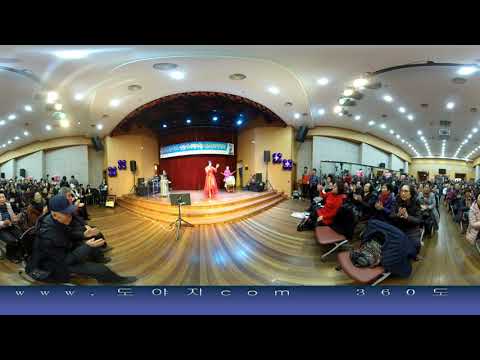This image is a 360-degree panoramic view of an indoor auditorium featuring a central stage approximately three steps high. The stage is framed by a deep red curtain at the back, and the surrounding walls are a light tan color with a hint of blue. The auditorium has a wood plank floor that adds a classic texture to the setting. On stage, there is a performer in a long, red dress standing near a music stand, with another performer positioned just behind her. The ceiling is white with recessed lighting that illuminates the room. The audience, which fills the auditorium, is seated in orderly rows of chairs, wearing a variety of mostly dark-colored clothing, and some individuals are even sporting hats. The image is bordered in black at the top and bottom, with a blue strip running across the bottom edge featuring text that includes "www dot [...] dot com" and the number "360," indicative of the panoramic format of the photo.